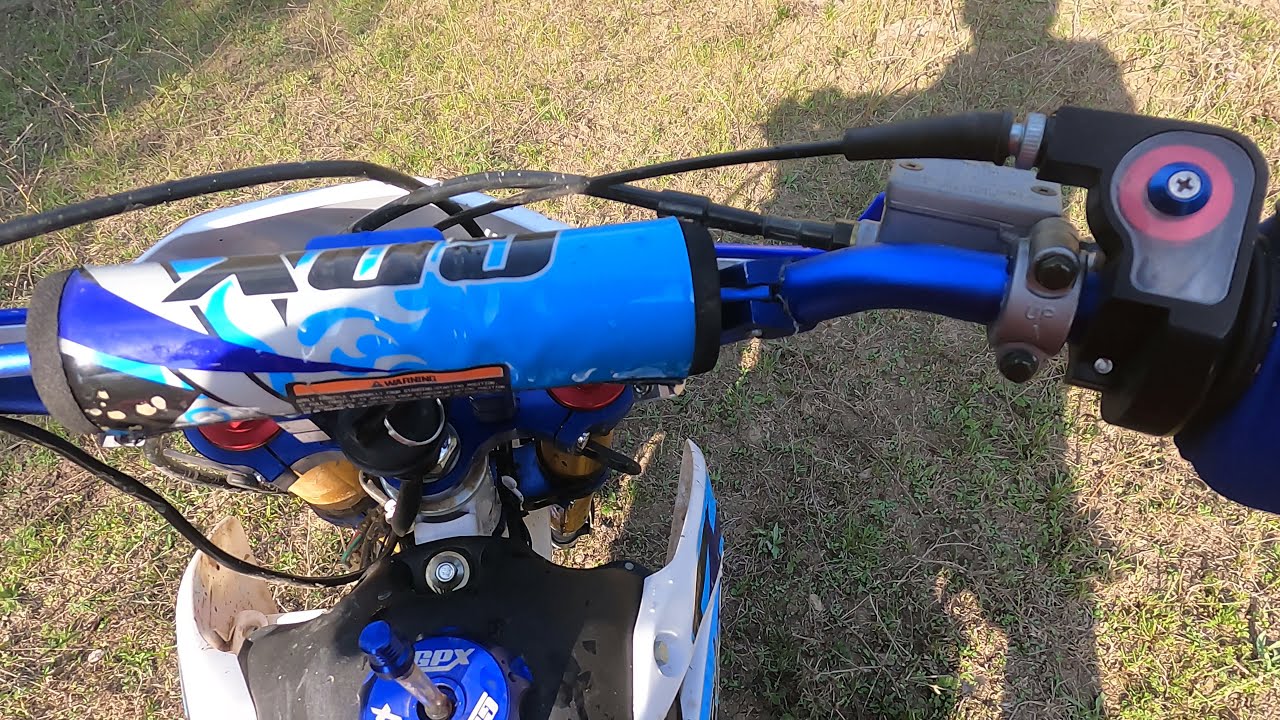This color photograph, captured in landscape orientation, presents a detailed, close-up view from a rider's perspective, possibly seated on a BMX bike or a dirt bike. The image appears to be taken with a GoPro camera mounted on the rider's helmet, offering a freeze-frame look over the handlebars. The handlebars, gleaming in a royal blue hue, are equipped with a blue cylindrical cushion featuring a dark blue swirl and black lettering. The left brake lever with accompanying cables is visible alongside the right grip being held by a gloved hand, clad in blue. 

The bike's body is predominantly white, adorned with blue graphical stickers. Below, the ground is a mixture of sparse, dried grass and dirt, suggesting a dry and weedy terrain. The rider's shadow stretches from the bottom of the image towards the upper right corner, indicating that the sun is positioned behind the rider, shining from the left shoulder. This composition captures the essence of a sunny outdoor scene, embodying the thrill and realism of an active ride.